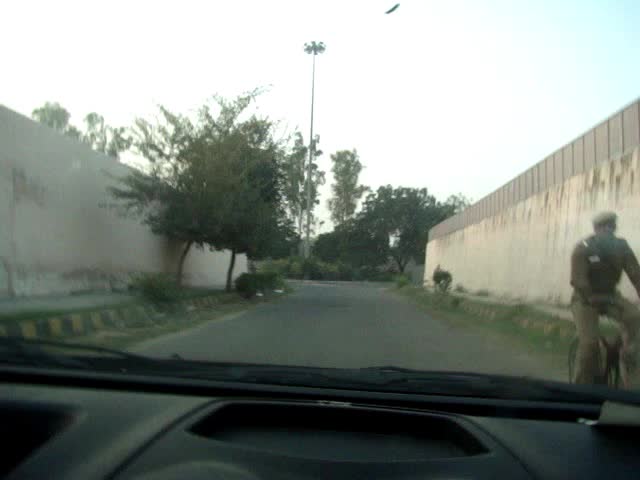Taken from inside a vehicle, the image showcases the dark gray dashboard and black windshield wipers prominently in the foreground. On the left side of the vehicle, a man on a bicycle is captured mid-motion, dressed in a military-style uniform consisting of khaki pants and a darker-colored top. He also wears a hat that completes his uniformed appearance. The scene outside includes a scraggly-looking tree with green leaves to one side and patchy, darker green grass on the other. A sidewalk runs adjacent to the street, leading past a gray concrete wall topped with a brown cap on one side, and another gray stone wall without a top on the opposite side. The curb near the stone wall features distinctive yellow and black paint markings. Further down the street, a light post and additional trees are visible, framing the urban landscape.